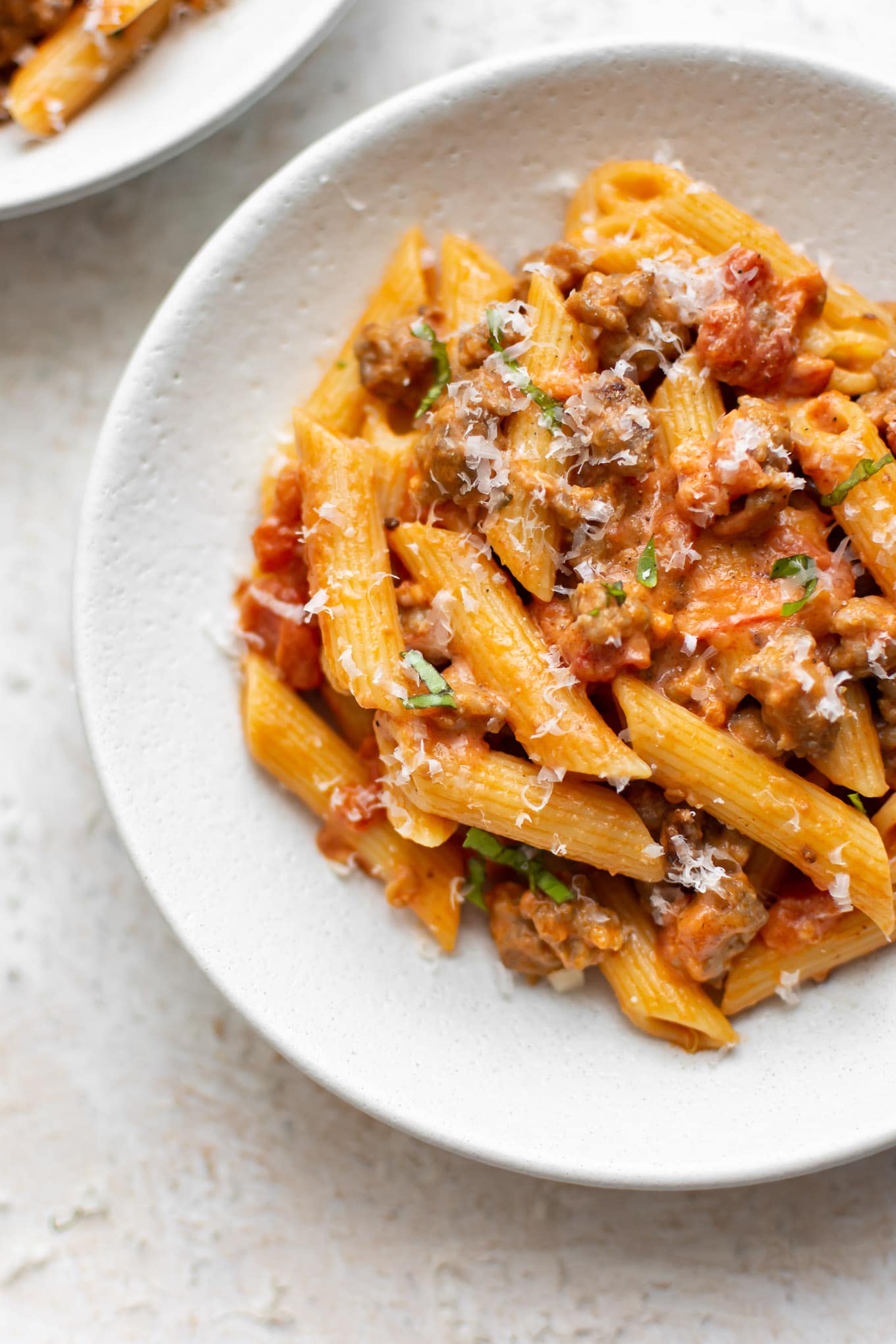The image is a top-view photograph of a white ceramic bowl filled with penne pasta, served in a red tomato-based sauce mixed with ground meat, most likely beef or possibly sausage. The sauce also contains distinct chunks of tomato. Generously sprinkled over the pasta are shreds of white parmesan cheese and scattered green herbs, potentially basil. The white marble countertop adds a clean, sophisticated backdrop. In the upper left corner, a small portion of a similar pasta dish is visible, suggesting a shared meal. The creamy appearance and fresh presentation of the pasta make it look immensely appetizing and delicious.